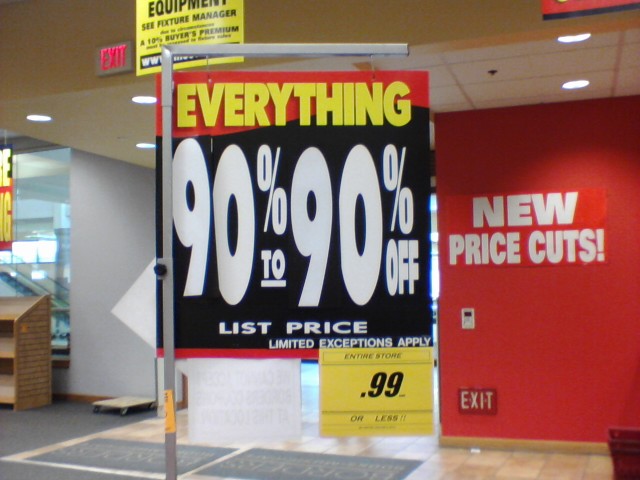A photograph taken inside a store captures a somewhat confusing sale sign. The sign reads "Everything 90 to 90% off," which doesn't quite make any sense. It's apparent that the sign has been altered, as the "90" on the left side has a "9" placed over what appears to be the original number, possibly "50" or another figure. This suggests that the store might be desperately trying to advertise an ongoing or final clearance sale. In the background, the right side of the image shows a red-painted wall with the phrase "New Price Cuts" displayed prominently.